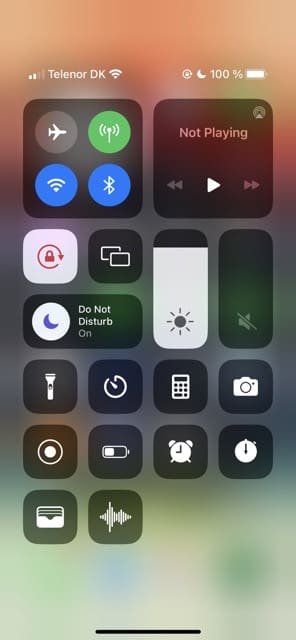A detailed and cleaned-up version of the caption could be:

"This image showcases the settings drawer of a smartphone, accessible by swiping down from the top of the screen. The cellular network is Telenor DK, and the battery is fully charged at 100%. The settings drawer includes various essential toggles and controls: Airplane Mode, Wi-Fi, Bluetooth, and a radio signal button, which may be for picking up radio signals. There is also a music control box that allows you to play, pause, skip, or reverse tracks. Additional options include a lock phone button, a Do Not Disturb toggle, brightness and volume controls, a flashlight, calculator, reminders, photo or camera app, timer, stopwatch, battery indicator, and several other icons with unspecified functions. This comprehensive drawer provides quick access to the phone's key settings and tools."